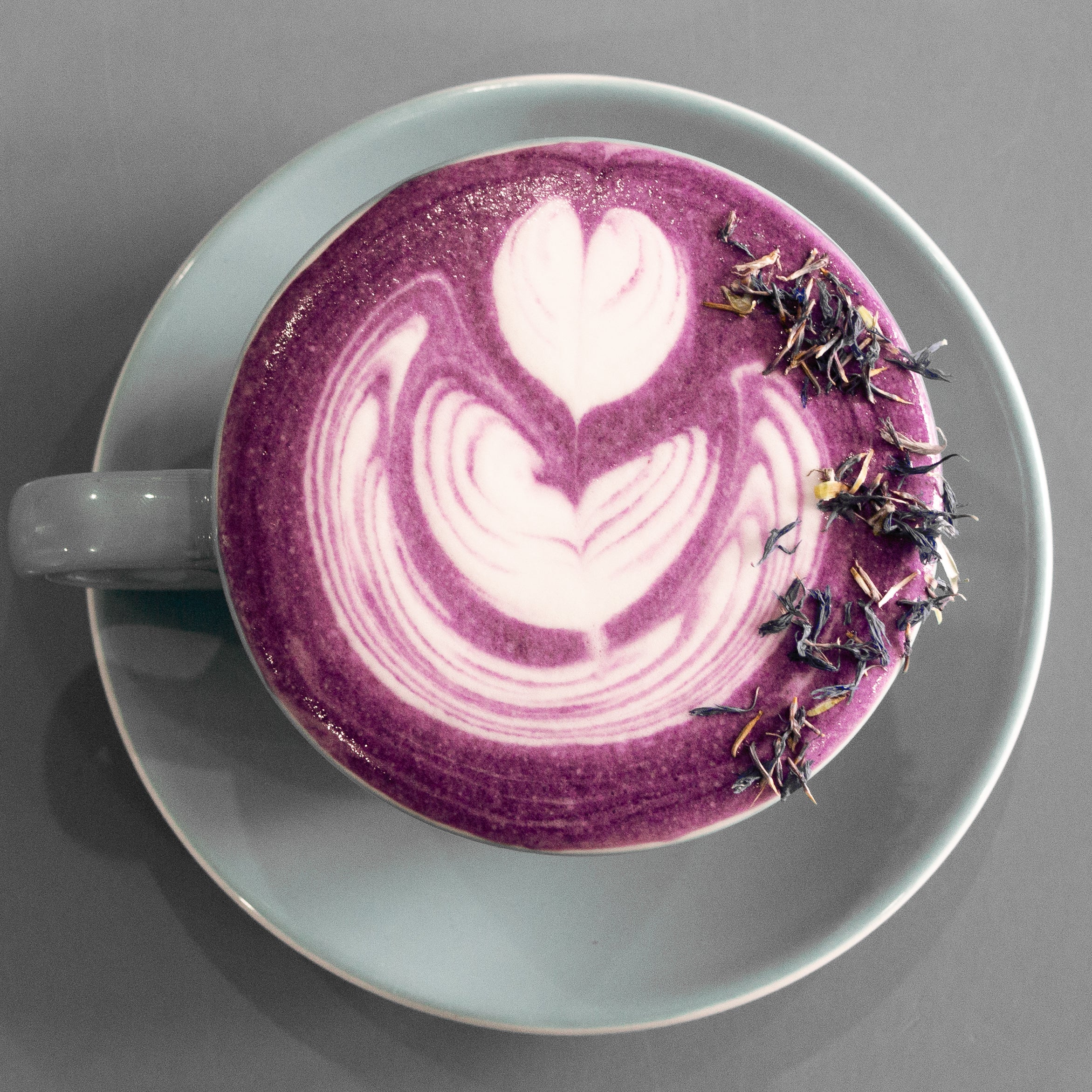This image showcases a beautifully crafted lavender coffee served in an off-white cup with a matching saucer, viewed from a top-down perspective. The coffee itself is a striking purple hue, which transitions from a darker shade at the edges to a lighter purple towards the center, blending seamlessly with the white cream. Atop the beverage rests an intricate cream floral design, resembling a heart or flower, created from the milk foam. The rim of the cup is garnished with dried lavender petals, adding a touch of elegance and complementing the vibrant purple of the drink. The handle of the cup is positioned to the left, featuring a round-edged design. The overall presentation highlights the artistic and appetizing appeal of this specialty lavender coffee.